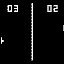This image is a tiny, square screen capture of what appears to be the game Pong, one of the earliest video games. The background is predominantly black. Dominating the center of the image is a vertical white line, which resembles a net in a game of electronic tennis. In the top left corner, the number "03" is displayed, while "02" is shown in the top right corner, possibly indicating the scores. The left side of the screen features a small vertical white rectangle near the bottom, with a white square or dot adjacent to it. On the right side, a similar small vertical white rectangle is positioned just above the center. The simplicity of the design aligns with the aesthetic of Pong, making it likely that this is an early iteration or representation of the game.